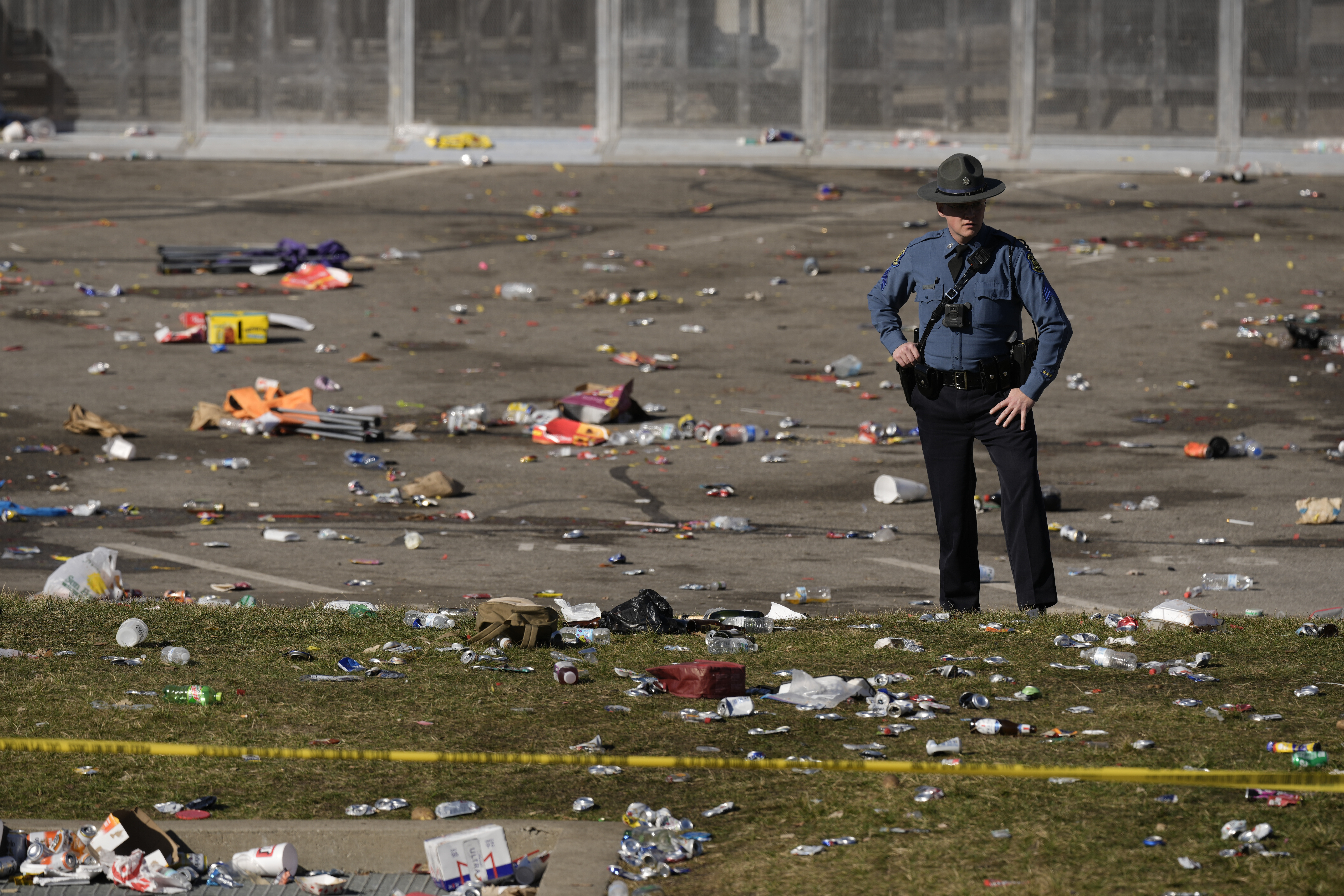The image portrays a disheartening scene at what appears to be an event aftermath, possibly the Kansas City Parade shooting. In the foreground, a police officer or state trooper, characterized by a gray, broad-brimmed hat, a blue button-down shirt, black pants, and a radio, stands amidst the debris. The officer, with hands on hips and a disgusted expression, gazes over the vast expanse of litter, which includes styrofoam cups, bottles, papers, and fast-food bags from Chick-fil-A or Target. The rubbish sprawls across the entire parking lot and adjacent grass, demarcated by "Police Do Not Cross" yellow tape. A mesh fence borders the scene in the background, contributing to the fenced-in, forlorn atmosphere. The event's aftermath, visible through scattered folding chairs and the overwhelming trash, hints at a large gathering or disturbance. Additionally, a large building with expansive glass windows looms behind the officer, adding to the desolation of the setting. The pavement is punctuated by the border separating it from the trash-strewn grass, portraying the stark division between order and chaos.